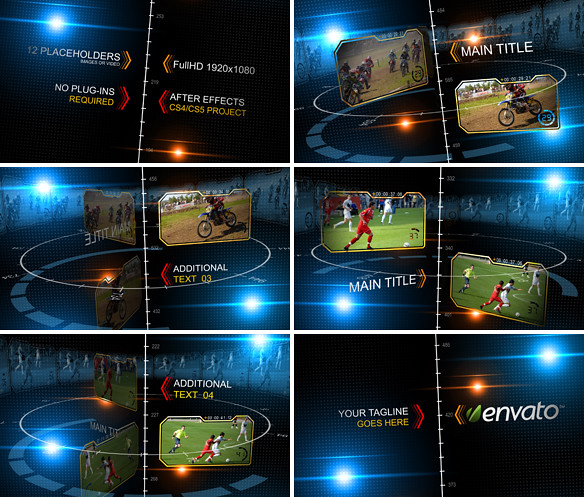The image is a structured layout, divided into six even sections arranged in two columns of three rows. Each section is further split into two parts by a white line, with jagged white lines separating images and text. In the top left section, text reads, "12 placeholders, no plugins required" on one side, and "Full HD 1920 x 1080" with "After Effects" on the other. The top right section features dirt bikes, with the text "main title" beside an image of a person riding a bike. The middle left section combines "Additional Text 03" with an image of a biker, while the middle right showcases soccer players and another image of people playing football. The bottom left segment has two blurred pictures of football players, accompanied by the description "Additional Text 04" and a vivid football scene. The bottom right section states, "your tagline goes here" next to the Envato logo, a green abstract leaf. These visual elements suggest the template is for a customizable HD advertisement, indicating features and placeholders for various sports imagery.